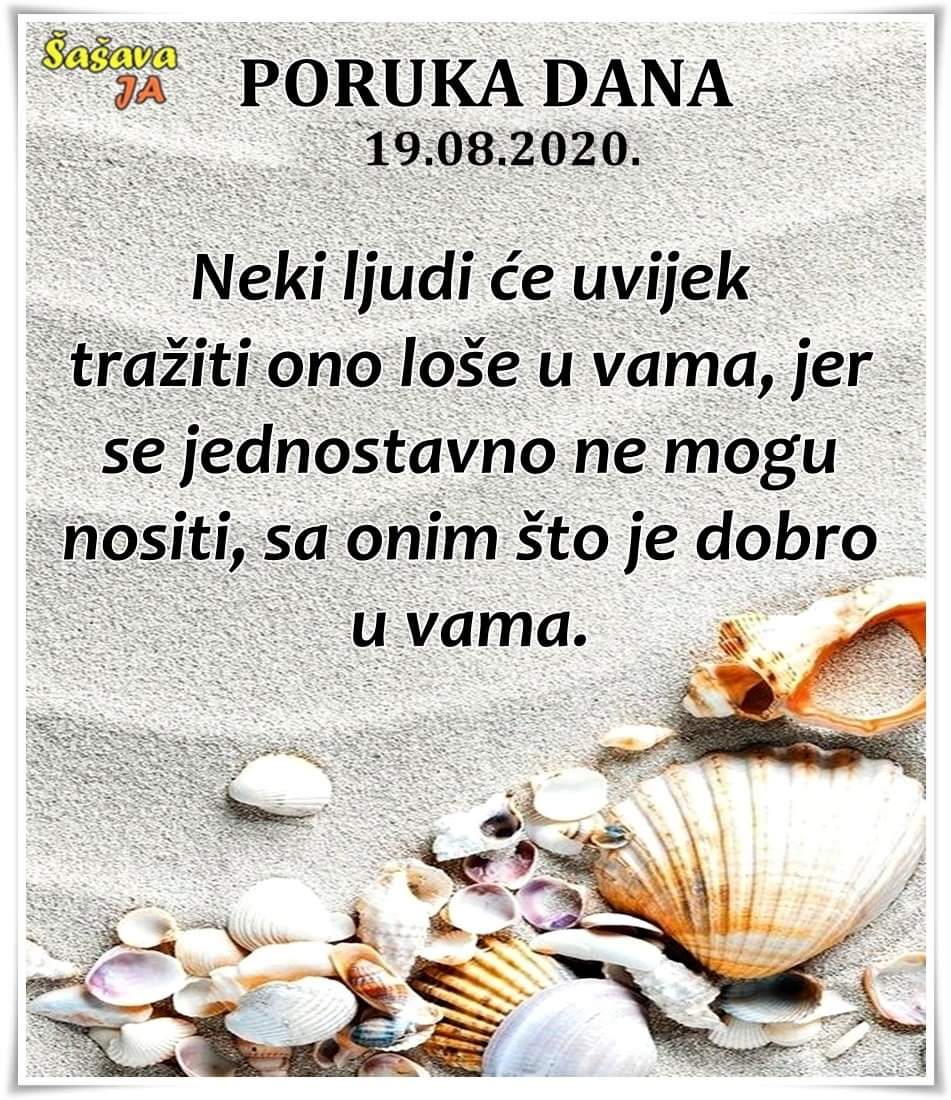The image features an inspirational text in Polish, set against a serene beach scene. The background is composed of fine, grayish-white sand with subtle waves. Seashells of various types, sizes, and colors—ranging from white and purple to shades of dark orange—form an angular flow from the bottom left to the upper right corner. At the very top of the vertical image, the title "Parooka Dana, 19-08-2020" is written in black text, followed by a paragraph in the same font in the center of the image. The black text of this paragraph reads "S-I-T-I-S-A-O-N-I-M-S-T-O-J-E-DOBRO-U-VAMA." In the top left, there are strings of yellow and orange text which read "S-A-S-A-V-A" and "J-A" respectively, further embellishing the image. The neutral tone of the beach and the colorful assortment of seashells complement the textual elements, creating a tranquil and inspirational scene.